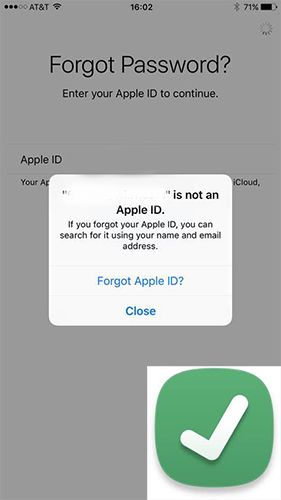A detailed caption for the image described could be:

"A smartphone screenshot showing a 'Forgot Password' prompt for an Apple ID. The screen has a semi-transparent gray overlay, with a white pop-up box displaying a message related to recovering the Apple ID. At the top of the screen, the status bar shows the AT&T network connection, a Wi-Fi signal, and a timestamp reading 16:02. The Bluetooth icon is disabled, and the battery level is at 71%. The main content of the screenshot includes a text field labeled 'Apple ID' and a message instructing the user to enter their Apple ID to continue. Below the pop-up box, a suggestion in black text reminds users that if they've forgotten their Apple ID, they can search for it using their name and email address, accompanied by a 'Forgot Apple ID' link in blue. In the bottom right corner, partially obscured by the gray overlay, there is a distinctive green oval icon with a white checkmark inside. This image clearly illustrates the step-by-step process for users to retrieve or reset their Apple ID password."